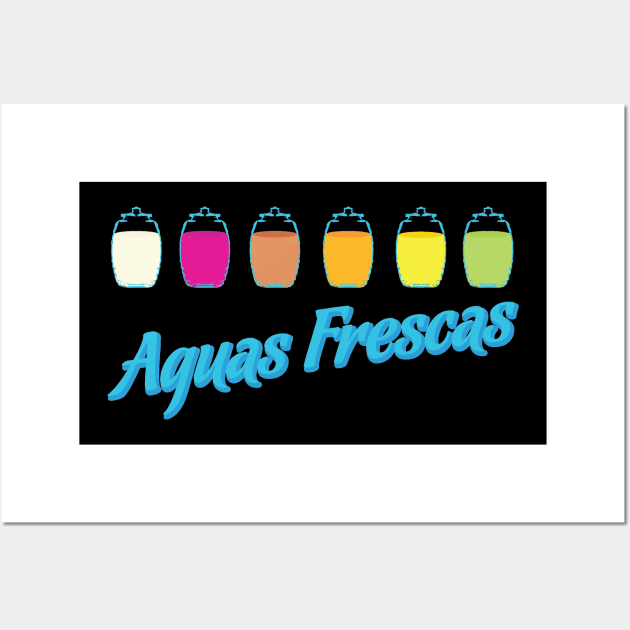This graphic design piece features a white rectangular frame centered within a light gray background. Inside the white frame, there is a smaller, longer black rectangle that acts as the backdrop. At the top of this black section, six jar-like containers with small stopper caps are displayed. Each jar is partially filled with liquids of distinct colors: from left to right, they are white, purple, pinkish-red, orange, bright yellow, and light green. These jars form a gentle upward diagonal from left to right. Beneath the jars, in large, light blue lettering, the title "Aguas Frescas" stands out prominently against the black background.